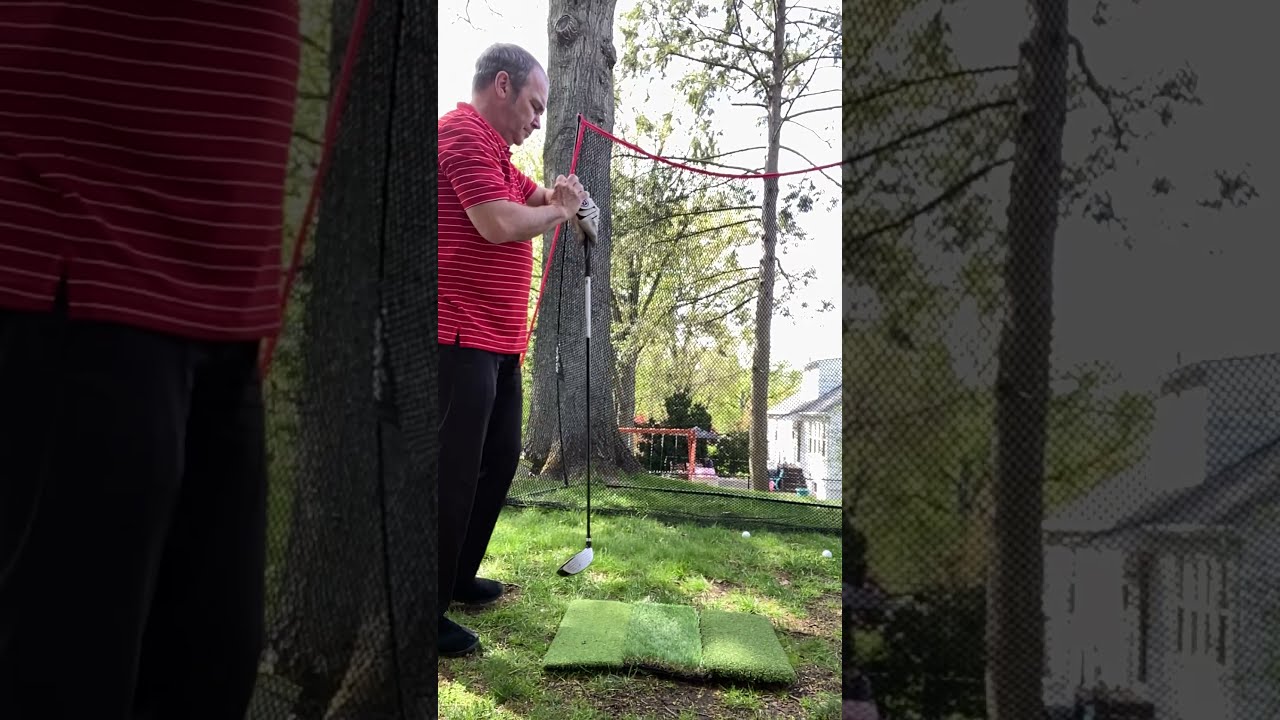In the photograph, an older white man, likely in his early 50s, is seen practicing golf in his backyard. He is adjusting something on his watch while holding a black golf club. The man is dressed in a short-sleeved red shirt with white horizontal stripes, black pants, and black shoes. He stands under the shade of a tree, and in front of him is a small putting green set on an actual grass lawn. The background reveals two white golf balls on the grass and a black netting likely intended to catch stray golf balls. Surrounding the scene are some trees, a house, and what appears to be a children's swing set. The image is set on a sunny day, possibly in the evening, indicated by the shadows. The overall composition features the main subject in a portrait mode centered against a lighter landscape version of the same scene. The man is alone, engrossed in his golfing practice.